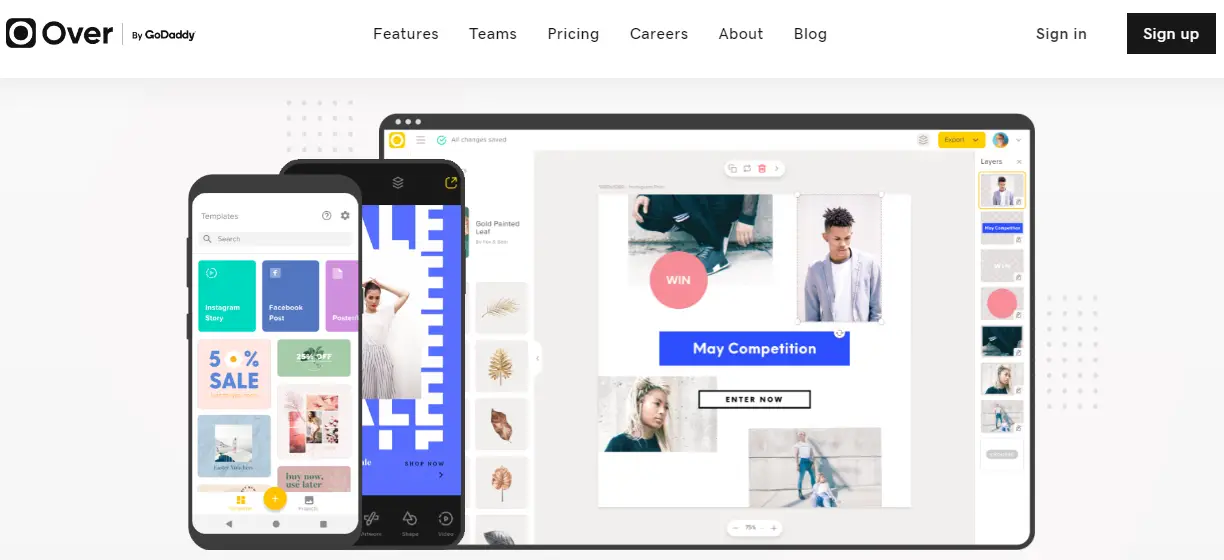This is a detailed and descriptive cleaned-up caption for the home screen of a website:

The top section of the home screen features a white header that transitions into a light grayish hue, gradually becoming almost white as it extends downwards. Within the white header, there is a black square containing a white border, which encases a black circle. Adjacent to this icon, the word "over" is written in black, with the phrase "by GoDaddy" in smaller letters beneath it. About two inches to the right, the navigation menu includes the following black text links: Features, Team, Pricing, Careers, About, and Blog. Towards the top right corner, there is a black tab inscribed with "Sign Up" in white text, and to its left, the option to "Sign In" written in black.

The main content area, set against a blue background, features a central tablet illustration with a black border. The tablet screen displays a search bar along the side, informational text on the left, and several images on the right. Prominently centered on the tablet screen is a blue banner that reads "May Competition." Below this, various images are depicted, including a man, shoes, and a girl. Superimposed slightly to the left of the tablet is a smartphone illustration with a black border, displaying a blue screen with a large white "E" and "L," along with a white silhouette of a person in the middle. Further to the left, there is a smaller phone with a black border and white screen, showcasing numerous icons and listings.